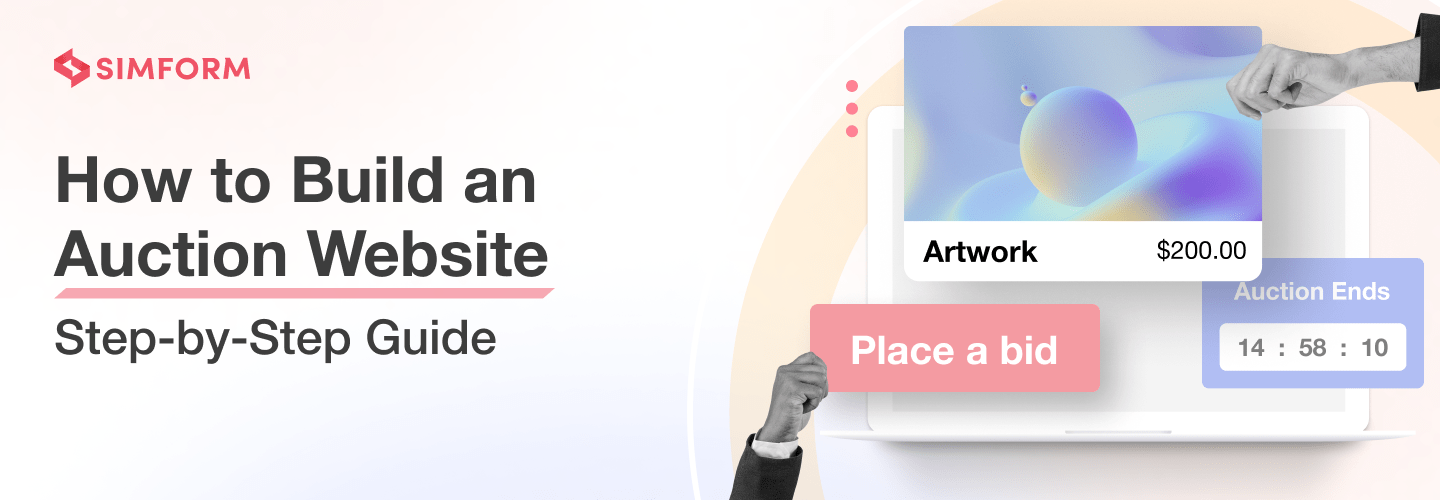The image appears to be an advertisement for Simform, featuring a step-by-step guide on how to build an auction website. It is set against a light, pinkish-white background with a circular pattern and includes various vividly colored elements. On the left-hand side, "Simform" is prominently displayed in a medium pink tone. Below this, in bold black text, it reads "How to Build an Auction Website," underlined by a long pink line, with the words "Step-by-Step Guide" underneath.

On the right-hand side of the image, there are two hands: one is holding a sign that says "Place a Bid" in white text on a pink background, while the other holds a piece of artwork labeled "Artwork" along with a "$200" price tag. The artwork depicts a sphere with a smaller sphere sticking out of it, set against a colorful yellow, green, and purple background. Just below this, a rectangular purple box contains the white text "Auction Ends 14-58-10." Three red dots further add to the design, enhancing the aesthetic appeal of this detailed and visually engaging advertisement.